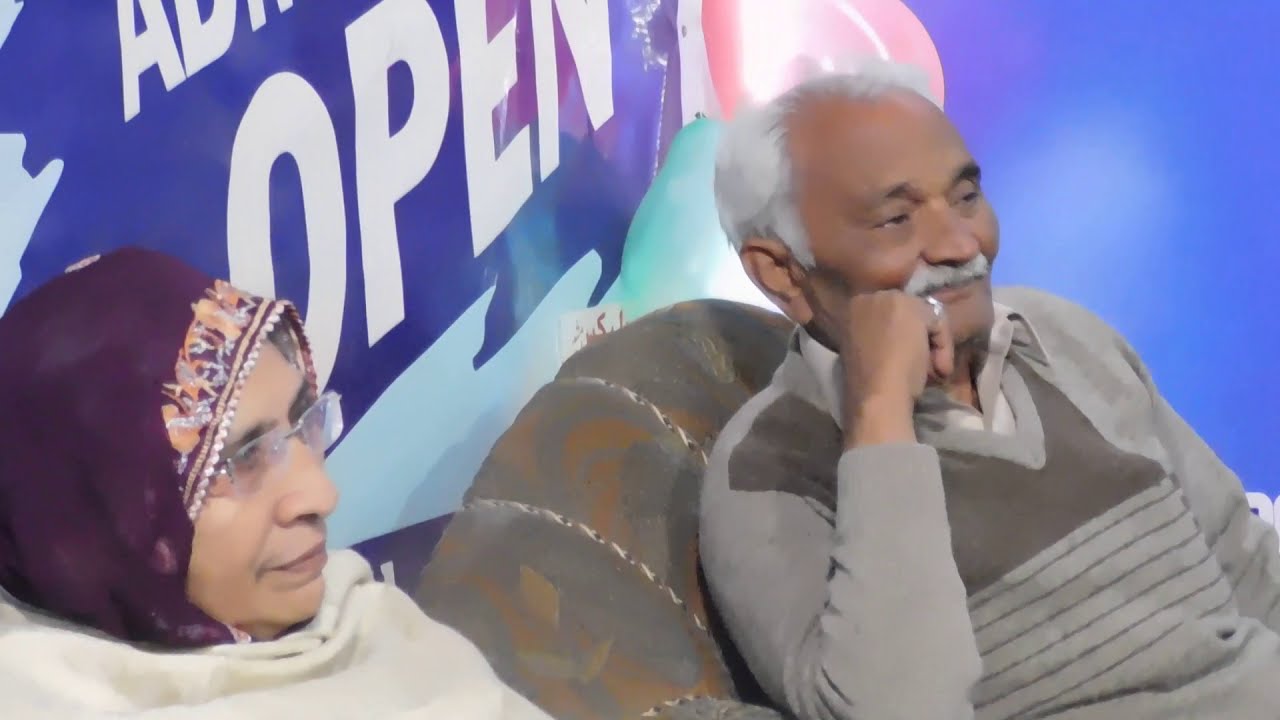The photograph captures a close-up of an older man and woman seated next to each other on a stage, possibly for a talk show or an interview. The background is vividly blue, with large white text spelling out "open" in a paint-splatter style. Behind them, ambiguous signage and possibly balloons suggest a festive or significant event. They are sitting on a couch; the woman, on the left, has olive-toned skin and wears glasses. She is draped in a white shawl and has a burgundy or dark maroon headscarf adorned with floral and lace trim, indicating an Islamic style of dress. She is visible only from the neck up. The man to her right has dark skin, a white balding head, a white mustache, and is dressed in a sweater with brown and gray stripes. He is also seated, but in a brown couch with embroidered stripes. Both appear to be listening attentively to something off-camera.